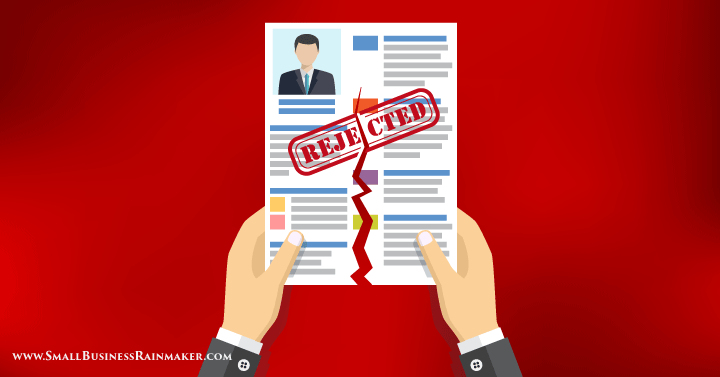This detailed digital illustration depicts a powerful image of rejection. At the center, a two-dimensional, faceless profile photo of a man appears on a white paper, resembling a resume. The man is dressed in a black suit with a blue tie. The document is adorned with blue section headings and gray horizontal lines, indicative of resume content. Across the resume, a large red "REJECTED" stamp stands out prominently. The paper is being torn apart by two human hands, each shown with thumbs in the front and fingers at the back, wearing white shirts and dark suits, implying a professional setting. The background is an intense, bright red, with variations of darker red shades. At the image's bottom, small white text reads "www.smallbusinessrainmaker.com," adding a subtle touch of context to the scene.